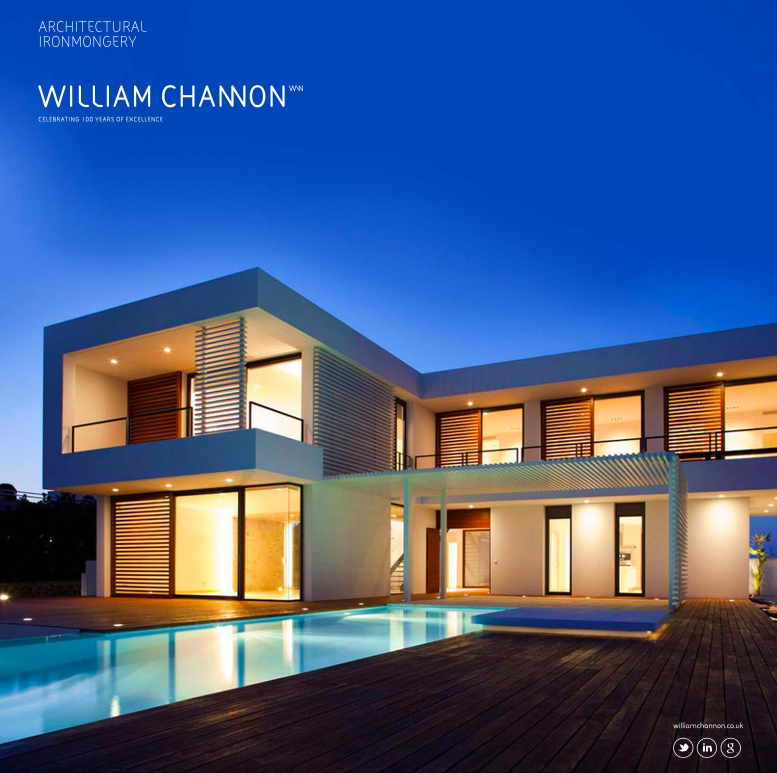The photo showcases a vertically rectangular, full-color image likely produced by an architectural firm, as noted by the white text in the upper left corner that reads "Architectural Ironmongery William Channon, celebrating 100 years of excellence." The image captures a modern, chic two-story building, potentially a high-end hotel or residence. The architecture is defined by its square, flat-roofed structure and numerous windows, all of which are brightly lit, suggesting either nighttime or dusk, with a deep blue, cloudless sky as the backdrop. The lower part of the image features a well-appointed wooden deck and a glowing swimming pool centrally positioned. Additionally, there's a mat on the deck and what appears to be a hot tub cover with a blue top on the right side of the pool. The area is enveloped in both natural and artificial lighting, highlighting the sophisticated design of the building and its inviting outdoor amenities. Logos for Twitter, Google, and another platform are also visible in the lower right corner, adding to the modern aesthetic of the scene.